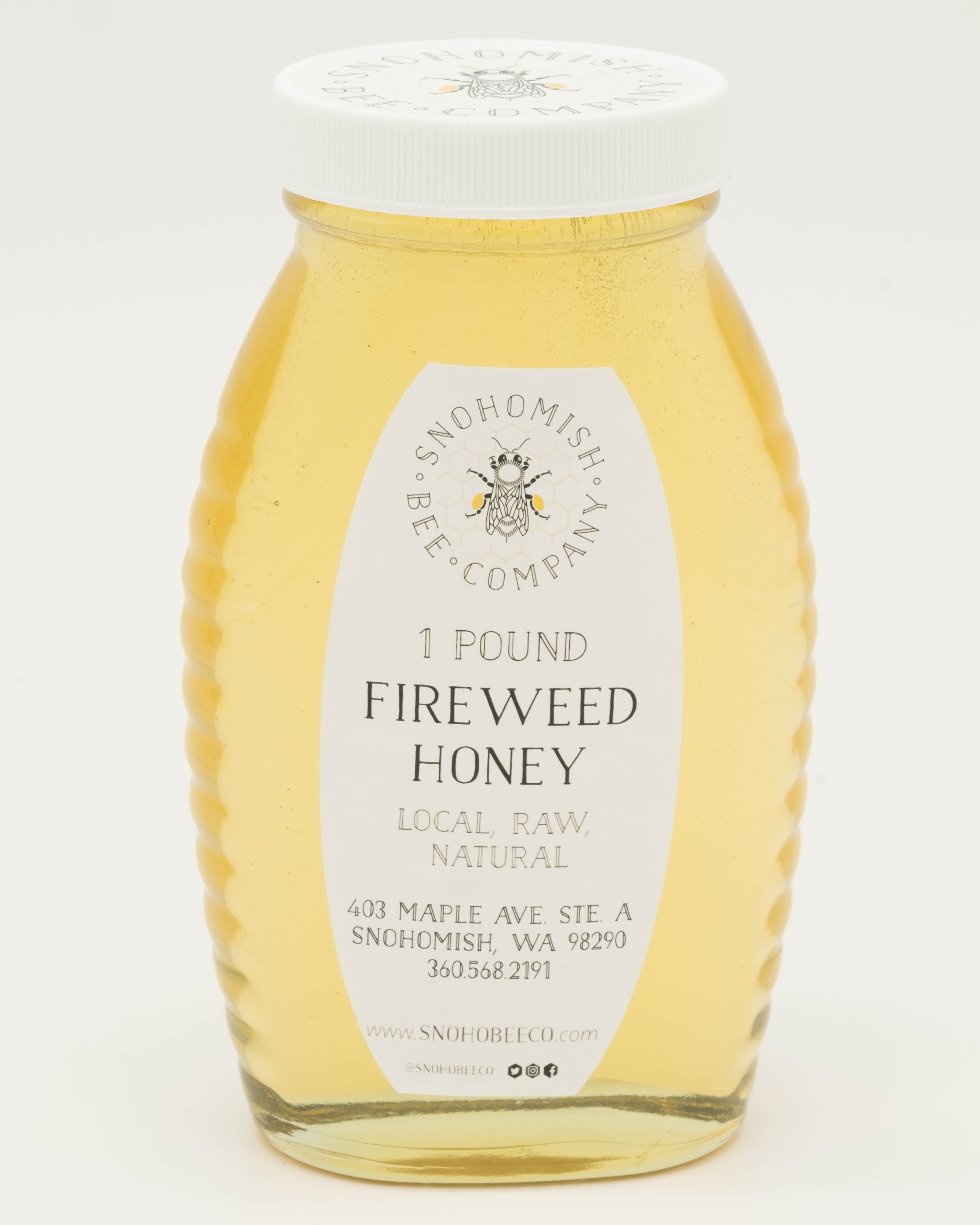This image depicts a clear, golden-colored jar of fireweed honey from Snohomish Bee Company. The jar features a distinct football-like shape with ribs along the sides and a white plastic cap. Centered on the cap is an illustration of a bee with text curving around it. The oval-shaped white label on the front includes a detailed drawing of a bee, notably with pollen on its legs. Surrounding the bee, it reads "Snohomish Bee Company," with "Fireweed Honey, Local, Raw, Natural" prominently displayed beneath. The jar contains one pound of honey and provides additional details at the bottom of the label: "403 Maple Avenue, Suite A, Snohomish, Washington, 98290," followed by a phone number, "360-568-2191," and the website "snohobco.com." The overall presentation emphasizes the natural and local essence of the honey, reflecting its artisanal origins. Social media symbols and faint additional text can be seen under the URL, adding a modern touch to this classic product.